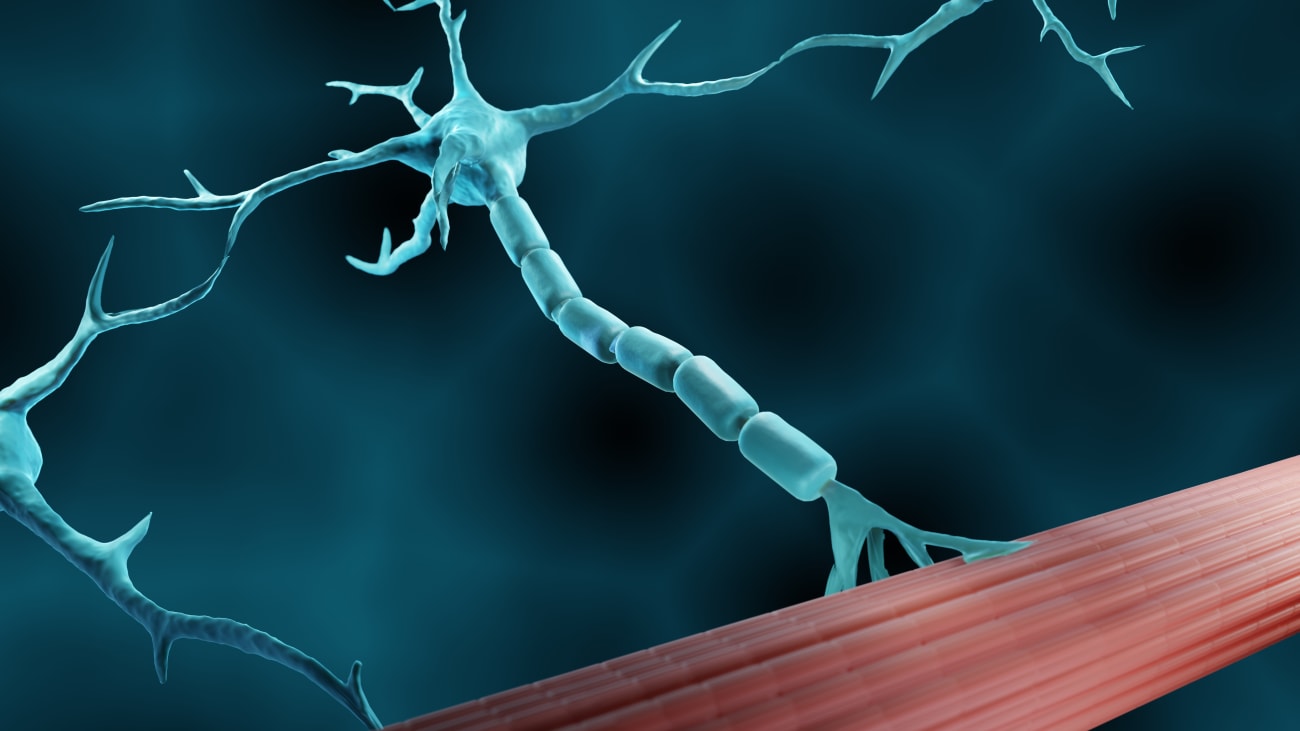The image depicts a computer-generated or digitally created artwork, possibly representing a biological entity on a cellular level. Set against a dark, somewhat teal-green and black background, the focus is on an intricate structure in the lower right-hand corner. This structure resembles a smooth, red, segmented branch or a long, red tube that extends diagonally across the bottom of the image. Attached to this red element is a lighter teal-green or blue object, which appears to be a round nucleus-like shape. From this central nucleus-like structure, vein-like or tendril-like extensions radiate outward in all directions, with thicker segments at the bottom transitioning to thinner ones at the top. These tendrils create a network as they connect to other similar round shapes. The background, although vague and faded, includes dark patches and blurred blue and black spots, enhancing the focus on the central nerve cell or neuron-like connection. This detailed composition suggests it might serve as a medical visual aid or an artistic representation of microscopic biological connections.